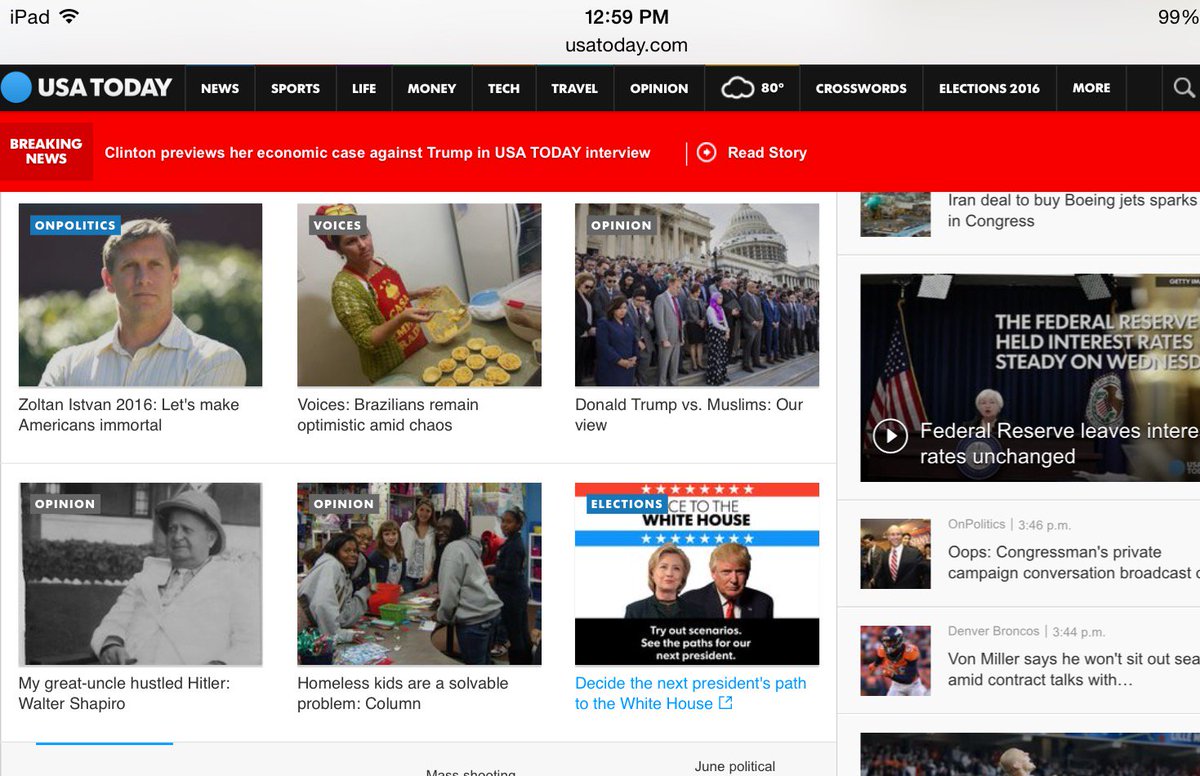The image captures a screenshot of the Apple website displayed on an iPad, as indicated by the "iPad" label in the upper left-hand corner next to a full Wi-Fi icon and a time display of 12:59 p.m. Below the time, the URL "ustoday.com" is prominently shown. On the upper right-hand corner, the battery status shows 99% charged. The background of the address bar is a light gray.

Beneath this, there's a black banner featuring the text "U.S. Today" on the left, accompanied by a blue circle. To the right of the title, the menu options "News," "Sports," "Life," "Money," "Tech," "Travel," "Opinion," and "Crosswords" are displayed, followed by a weather summary indicating "80 degrees." Next in the sequence are "Elections 2016," "More," and a magnifying glass icon for search functions.

Below this black banner, a red banner runs across the width of the screen's left side, indicating "Breaking News" in a transparent box. The headline "Clinton previews her economic case against Trump in USA Today interview" is displayed, followed by a dividing line and the prompt "Read Story" accompanied by a circle with a dot to the left of it.

Further down, six smaller media images are displayed horizontally. The first image is labeled "On Politics" featuring Zoltan Istvan. The last one, which is highlighted, states "Decide the next President: Pay up to the White House" with images of Trump and Clinton. On the right side, the partly-visible text "Federal Reserve leaves interest rates unchanged" and a play button appears, displaying an image of Janet Yellen. There are also two partially visible articles underneath this section.